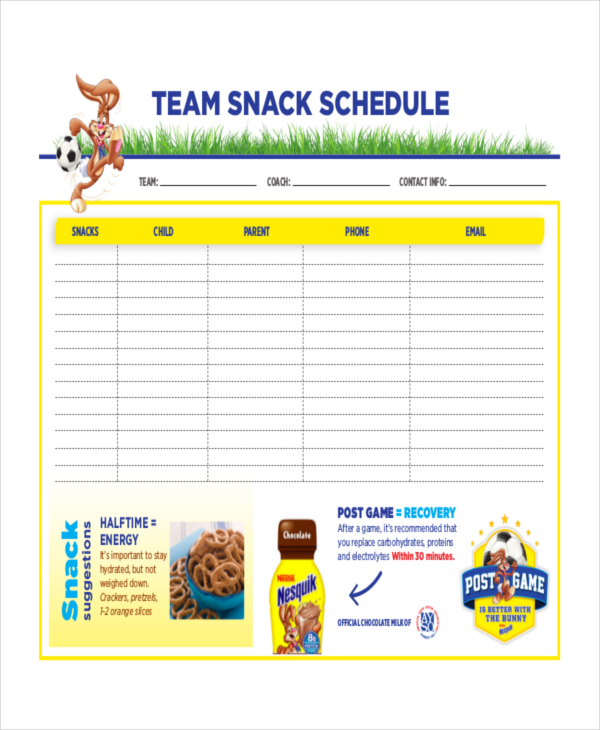This image features a detailed schedule form from Nestle Nesquik, ideal for organizing team snacks at Little League sporting events. At the top, in bold blue capital letters, "Team Snack Schedule" is prominently displayed. Just below this title, the beloved Nesquik brown rabbit mascot is illustrated kicking a soccer ball, with green blades of grass growing from a horizontal blue underline beneath him. 

The form is structured for easy input of team information, featuring sections labeled "Team," "Coach," and "Contact Info," each accompanied by horizontal lines for writing. The main body consists of a grid with headers in blue font on a yellow background, titled "Snacks," "Child," "Parent," "Phone," and "Email." This grid is laid out with dotted lines to fill in details for various entries.

At the bottom, a designated section offers insightful tips under "Snack Suggestions." It emphasizes "Halftime equals Energy" with pointers about staying hydrated without feeling weighed down, recommending snacks like crackers, pretzels, and 1-2 orange slices. Beside this advice, a photo shows a blue bowl filled with pretzels. Adjacent to the suggestions, a yellow bottle of Nesquik chocolate milk is highlighted under "Post Game equals Recovery." An accompanying note advises replenishing carbohydrates, proteins, and electrolytes within 30 minutes post-game. Further right, another emblem featuring the Nesquik rabbit with a soccer ball and yellow stars underscores that "Post Game is better with the bunny." 

The overall design is colorful, featuring a palette of white, blue, green, yellow, red, and light blue, resonating with the playful yet practical theme fitting for youth sports activities.